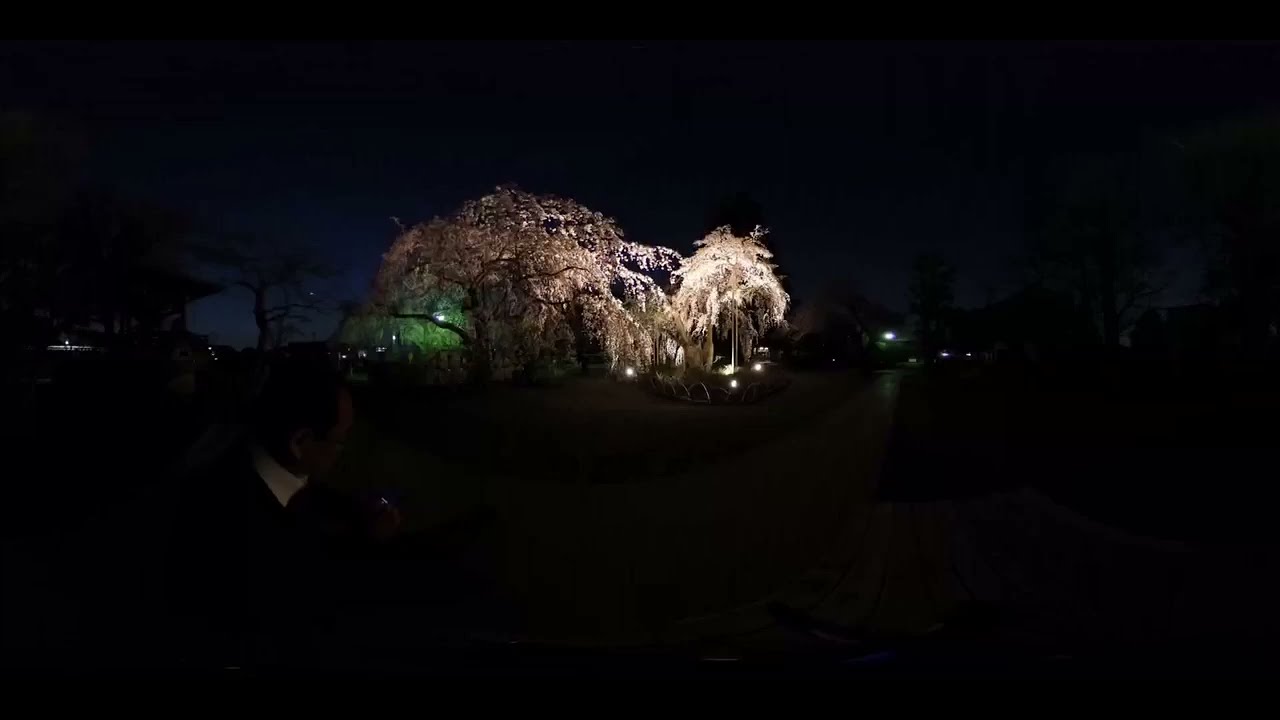In this nighttime panoramic photo taken in a park, a man with short black hair and glasses is seated on a wooden bench to the left, gazing at his smartphone. He is dressed in a white collared shirt under a red sweater and a dark brown jacket. His right leg is crossed comfortably over his left knee. The sky retains a hint of blue, indicating it isn't completely dark yet. 

The camera’s curved view reveals a U-shaped path that extends in front of the bench, leading to a patch of brownish grass and an array of large willow or sakura trees. These trees are illuminated with an array of colors, including shades of white, yellow, and green from lights positioned below them. To the right, more trees and buildings are faintly visible, bathed in green lights. A green gazebo can also be spotted in the distance. The serene setting captures the man engrossed in his phone, creating a calming and reflective atmosphere.